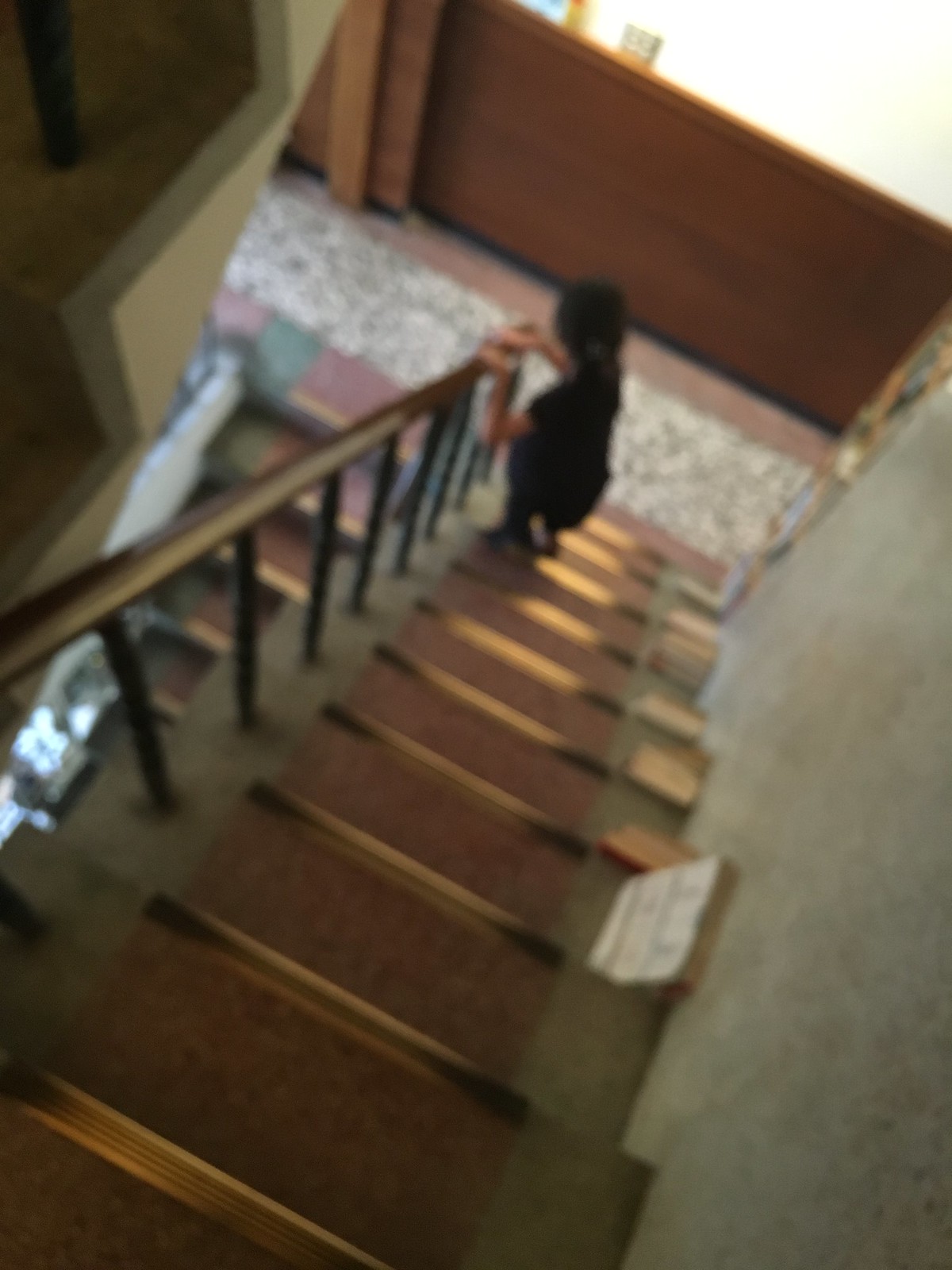This image captures a blurry photograph of an actual picture taken from a bird’s-eye view, showing a child walking down a flight of stairs. The perspective highlights the substantial height and numerous steps, suggesting the building has multiple floors. The child, dressed entirely in black with black hair, holds onto the banister with both hands. The stairwell features brown wainscoting along the walls and a window allowing sunlight to stream in. A red Oriental rug runner, adorned with a floral pattern in the middle and red trim, covers the wooden steps. Additionally, the steps have bands of metal across them. Given the details and decor, this setting likely depicts an institutional or commercial building rather than a private home.